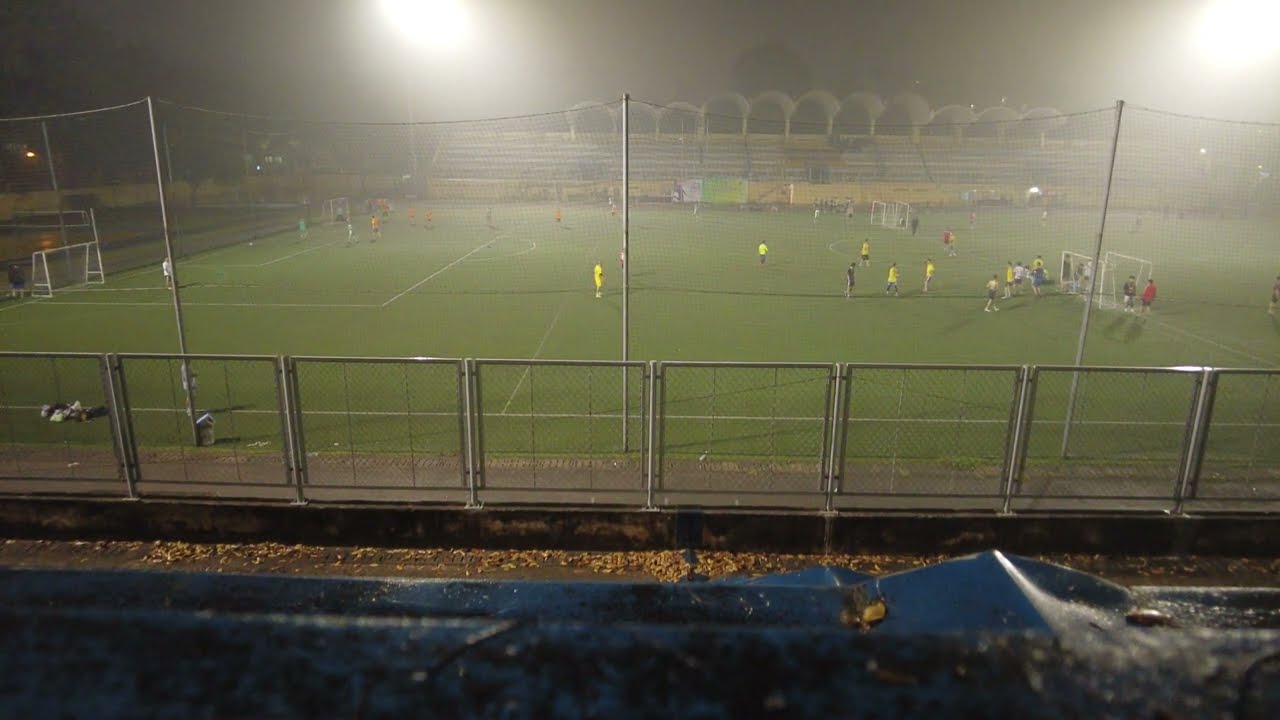The image captures a nighttime scene of a soccer stadium from the vantage point of the stands, likely the front row, as no rows are visible in front. The field, a verdant green adorned with precise white lines and goal posts at both ends, is flanked by fencing and enveloped in an atmospheric glow from fog lights positioned in the top corners. The pitch is divided into two areas where separate games are being played, with players predominantly donning red, orange, and yellow uniforms scattered across the field. Surrounding the stadium, the bleachers, visible through a silver gate and dotted with orange and brown leaves, appear damp, suggesting recent rain. On the opposite side, other structures and some illuminated buildings peek through the darkness, emphasizing the late hour of this vividly lit scene.